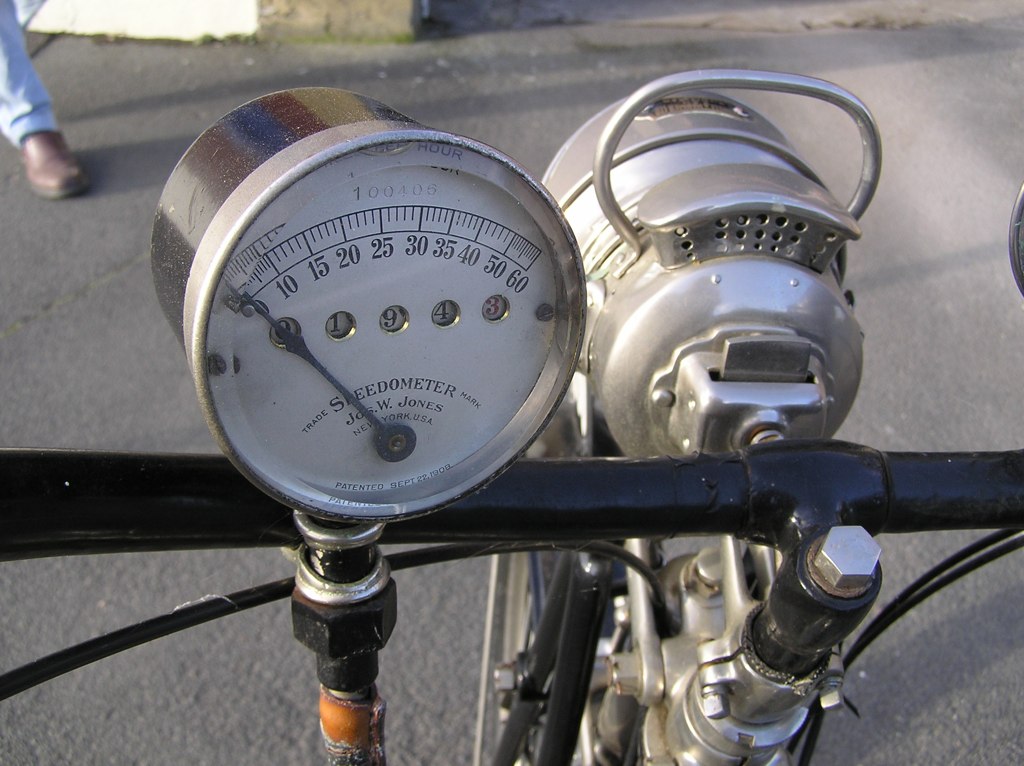This photograph features a meticulously detailed vintage motorcycle, potentially a three-wheeled model, though only a single front wheel is clearly visible. Prominently displayed is a heavy cast metal headlamp accompanied by black handlebars. Attached to the handlebars is an analog speedometer and odometer from the Jones company of New York, patented on September 22, 1908, with a range from zero to 60 miles per hour. The bolt securing the handlebars to the stem is clearly noticeable. Brake and/or clutch cables extend from both sides of the handlebars. In the upper left corner, the lower leg, foot, and boot of an individual are partially visible, adding a human element to the scene, which is set against a backdrop of a paved road.